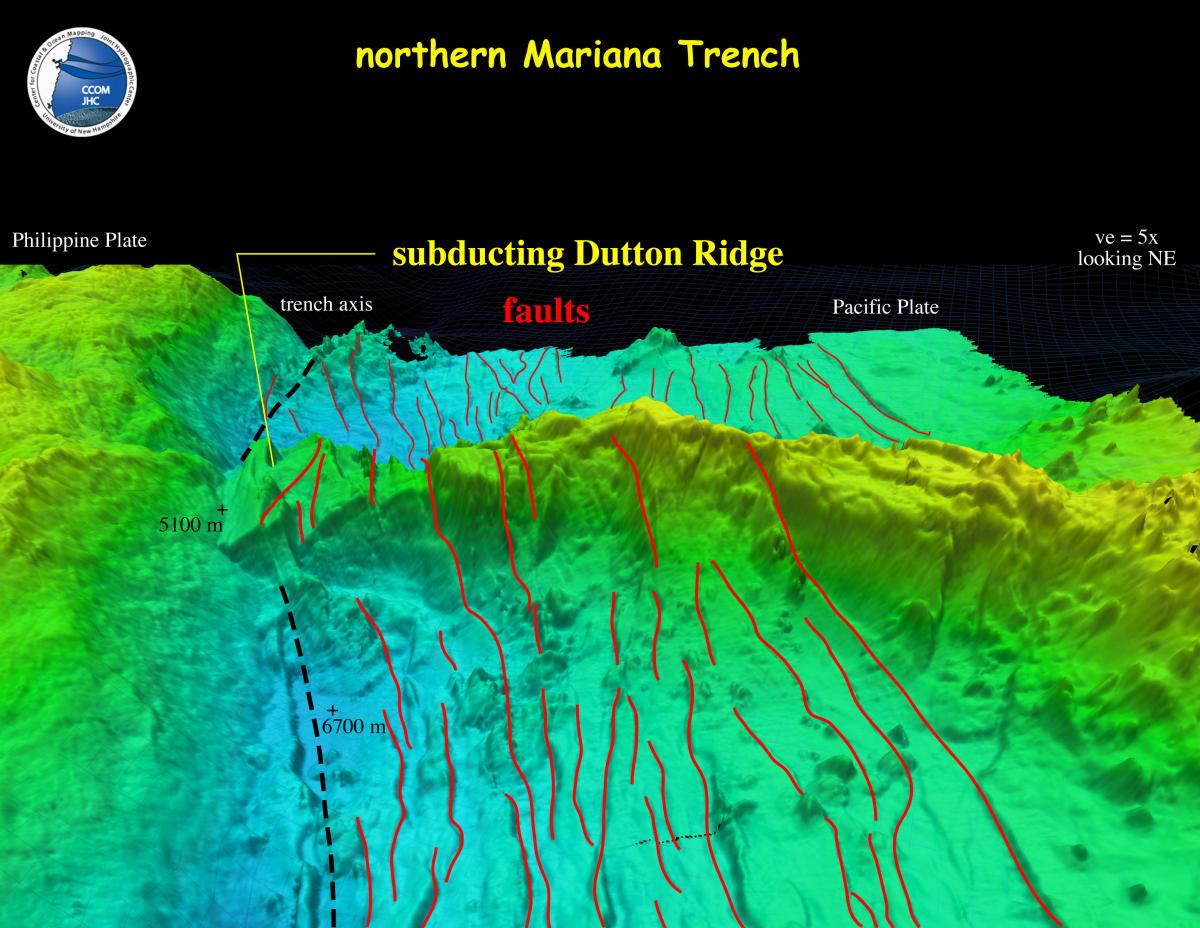The image is a detailed, scientific 3D topographical map of the Northern Mariana Trench, with labeled geological features and data magnified five times. In bold yellow letters, the caption "Northern Mariana Trench" sits at the top of the image, set against a black background. Beneath it, key features are labeled in white, including the "Philippine Plate" and the "Pacific Plate," which flank the "subducting Dutton Ridge." Fault lines, highlighted in red, traverse the center of the image, indicating areas of significant tectonic activity. A black dotted line marks the trench axis, with additional labels showing varying elevations, peaking at around 6,700 meters. This dynamic interaction between the Pacific and Philippine Plates is responsible for natural phenomena such as earthquakes, volcanic activity, and lava flows, explaining the recent surge in natural disasters in the region. The map includes a key in the right corner to aid interpretation of the different features.